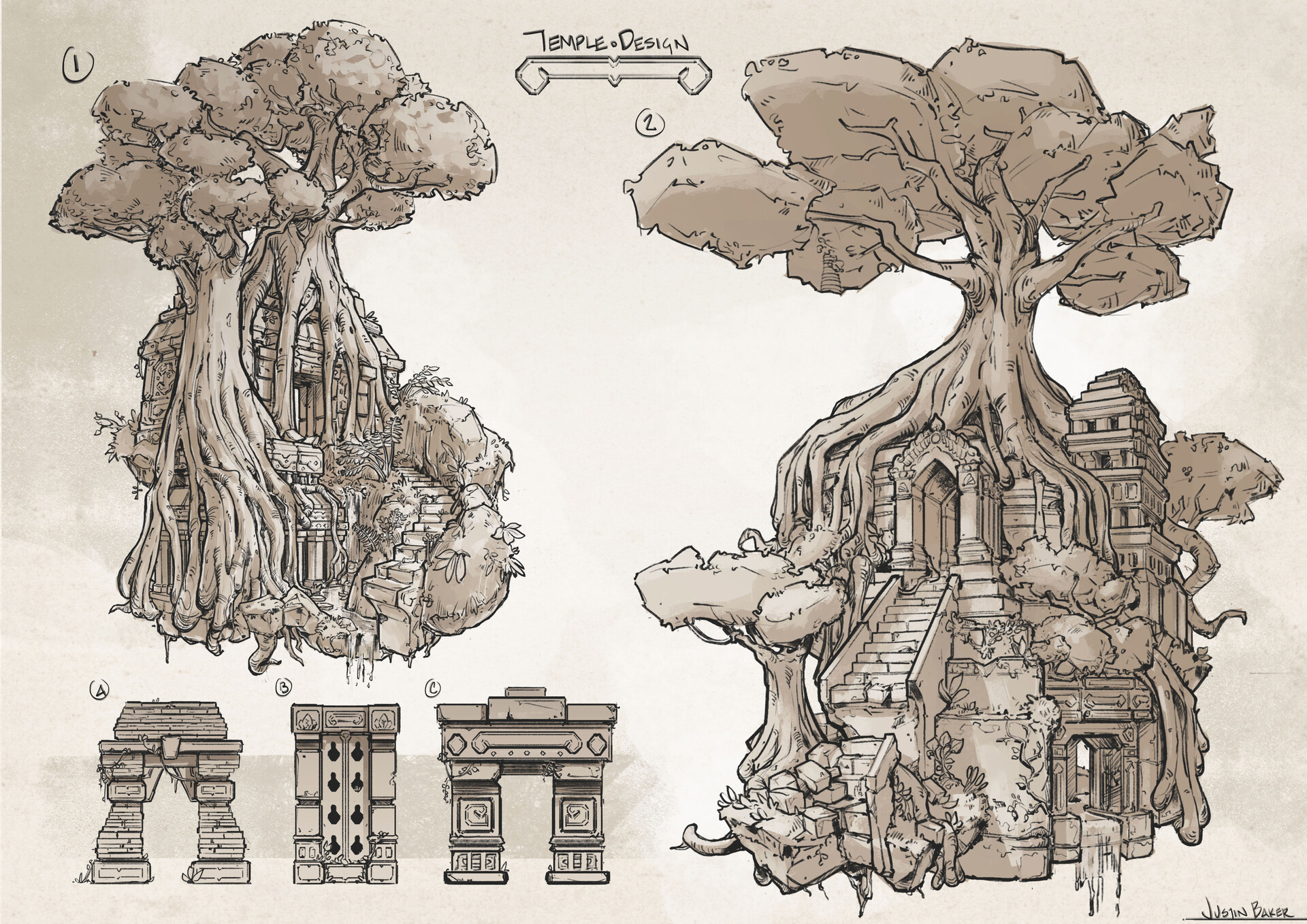This detailed digital line drawing titled "Temple Design" by Justin Baker, features a sacred, stone temple enveloped by the sprawling roots of a massive tree, as indicated by the text at the top, underlined. The image presents two main, large views of the temple, labeled one and two, depicting different angles. In drawing one, a staircase spirals towards the temple, while drawing two, the larger one, shows the tree's roots enveloping the temple, seemingly consuming it. Below these main views are three smaller sub-images, labeled A, B, and C, illustrating various sides, columns, and gateways of the temple, detailed without the tree. The entire illustration, rendered in a sepia theme, conveys an ancient, abandoned edifice, hidden, and almost overtaken by the natural growth surrounding it.